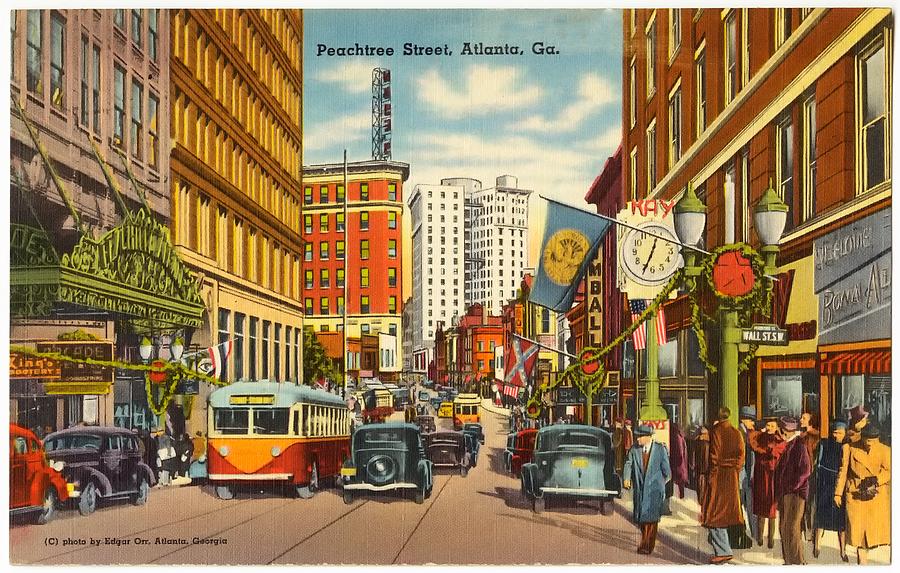This is a colorized illustration, possibly a vintage postcard, captioned "Peachtree Street, Atlanta, Georgia" at the top. Created by Edgar Orr of Atlanta, Georgia, it depicts a bustling city scene that appears to date back to the 1940s or 1950s. The street is alive with activity and features a variety of architectural styles among its tall buildings, including yellow, white, brown, and gray structures. Prominently, there's a building with a large clock and a theater with an elaborate gold sign that might say "arcade." On the left, there's a green sign for a movie theater, and a street sign reading "Wall Street SW" is visible on the right. 

The scene includes a mix of old-school cars, a red and orange city bus or trolley, and numerous pedestrians, many of whom are dressed in long trench coats. It's likely wintertime, as suggested by the Christmas decorations like wreaths and flags, including an American flag and another unidentified one. There are also signs for an arcade and a barber shop. The bottom left of the image bears the copyright mark, "photo by Edgar Orr, Atlanta, Georgia." The detailed and cartoonized nature of the illustration lends it a nostalgic, retro aesthetic, reminiscent of a bygone era.